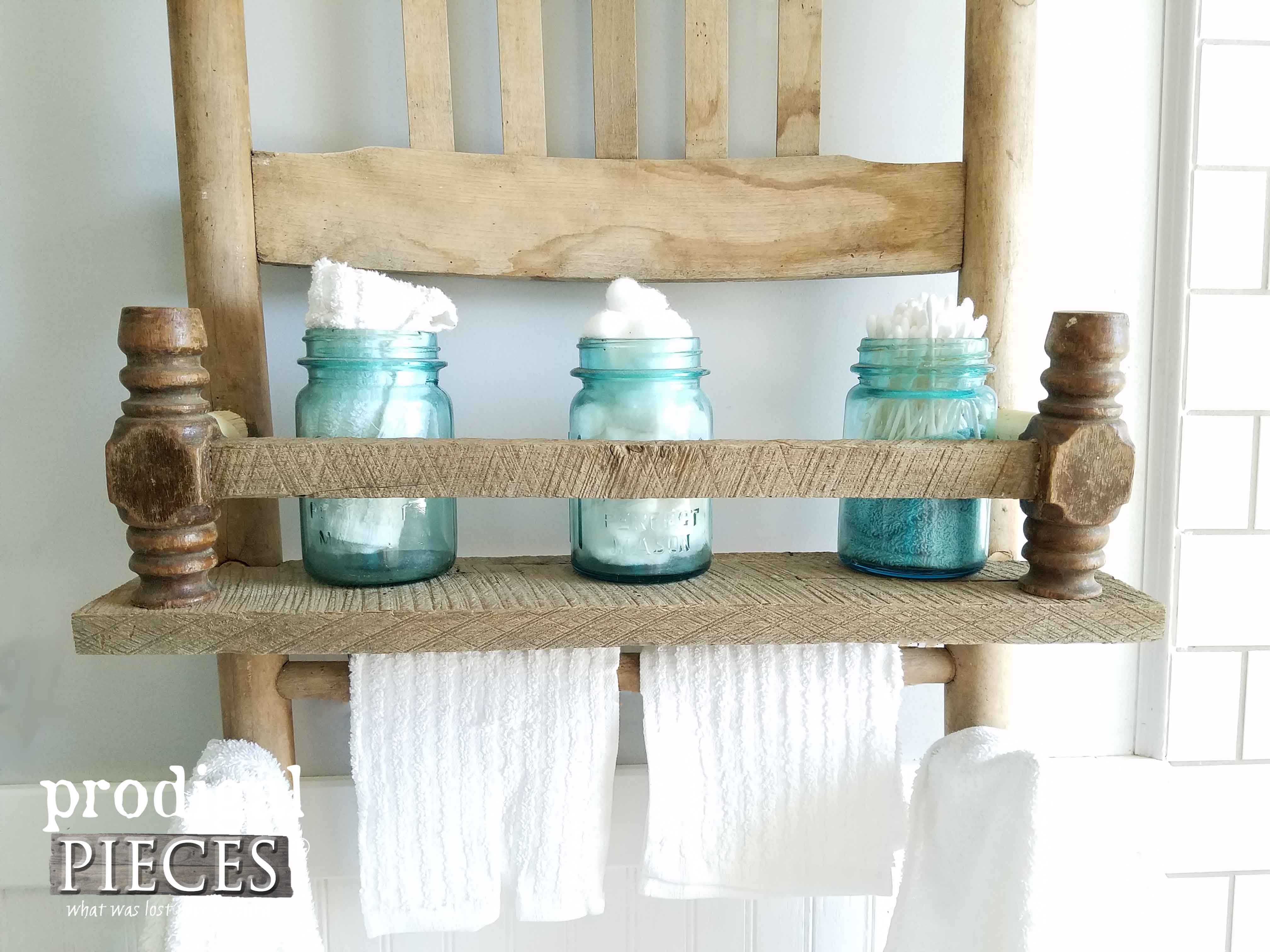This image appears to be an elegant advertisement for Prodigal Pieces, showcasing a beautifully crafted wooden bathroom shelf and towel rack. The wooden structure, reminiscent of a chair back with vertical slats and a horizontal top slat, exudes a charming, rustic aesthetic ideal for a country-style bathroom. The shelf, made of light wood, hosts three eye-catching aqua-colored mason jars. Each jar contains neatly organized white toiletries: cotton balls, q-tips, and washcloths, presenting a clean and serene look. Beneath the shelf, two white washcloths dangle from a wooden bar, flanked by hooks on either side that hold larger white towels. The simple, yet sophisticated arrangement is set against a backdrop of white tile, enhancing the ad's clean and inviting feel, making it perfect for a guest bathroom. The Prodigal Pieces brand name is subtly displayed in the bottom left corner, reinforcing the elegant design and quality of the products.